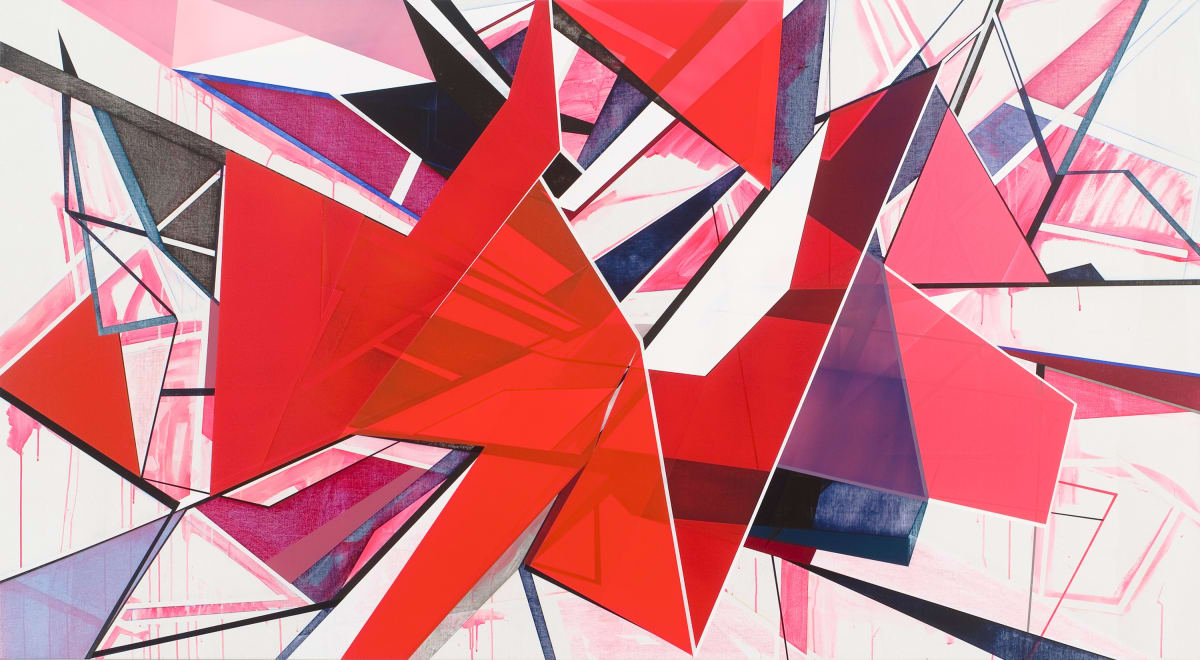This artwork, whether a drawing or painting, features a rich tapestry of abstract geometric shapes, predominantly in varying shades of red—from pastel red and lighter pinks to darker maroons and a blood-like ruby red. It skillfully integrates blues and blacks, with a background that darkens as shapes layer upon one another. The piece is a cacophony of overlapping and intersecting triangles, parallelograms, rectangles, and other undefined geometric forms, all appearing to converge towards the center. Lattice-like, dark and white lines intermittently bisect the composition, adding depth and creating a focal point within the vibrant spectrum of reds and blues. The overlapping shapes and intricate shading lend the work a dynamic, almost three-dimensional feel, making it a striking study in abstract form and color.